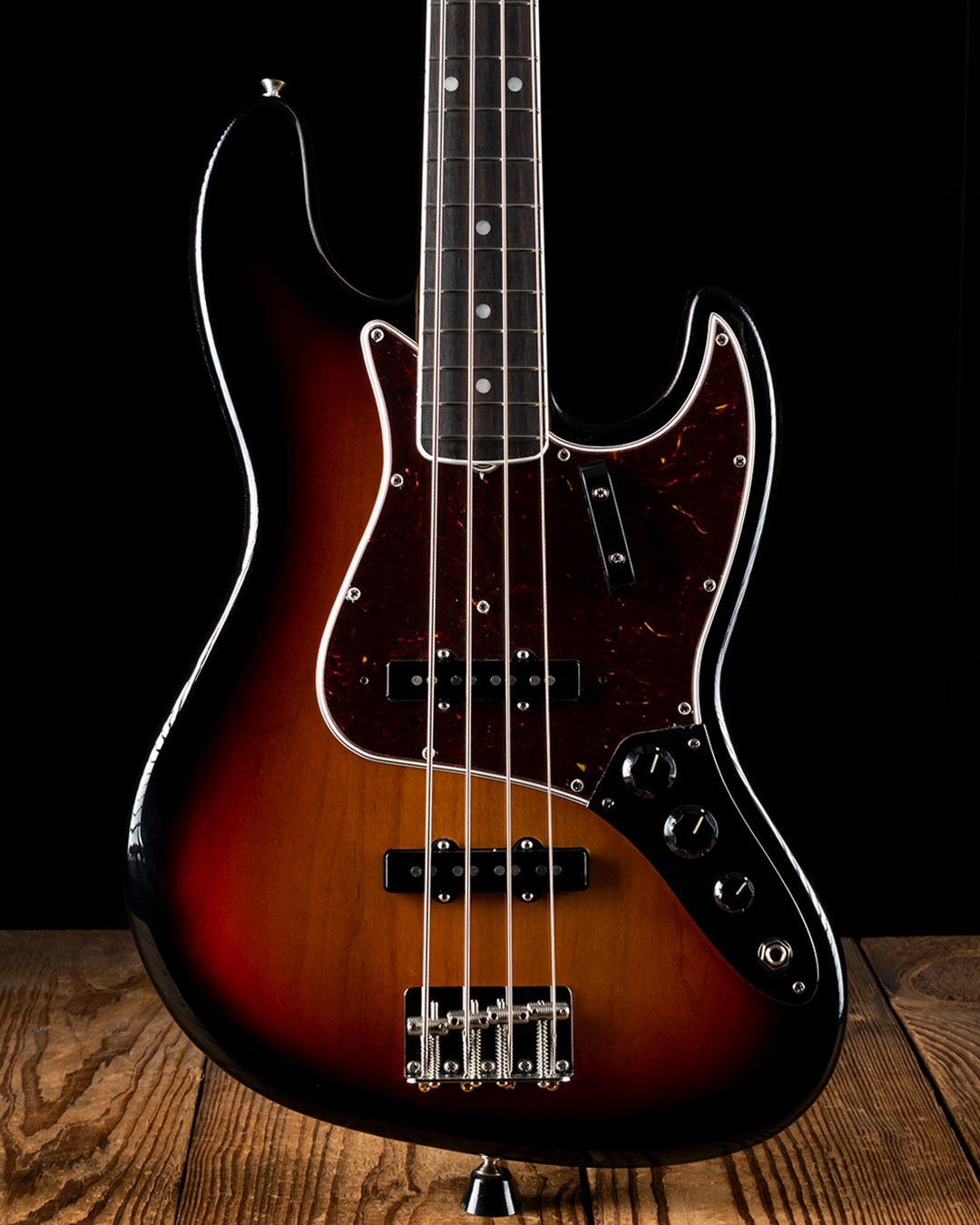This photograph centers on a distinctively styled electric guitar resting on the edge of a wooden table, set against a completely black background. The guitar, predominantly depicted from the base upwards, gets cropped out midway through its neck. Its body boasts a rich, brown hue transitioning to a nearly black center, accented by pure black edges. The guitar’s base is adorned with silvery metallic dials and buttons, and it features four gleaming white strings. Notably, there are three dials and a jack for plugging in an amp, along with visible screws highlighting its polished craftsmanship. The focal instrument slightly suggests it might be a bass guitar due to its four strings. The juxtaposition of the wooden surface and the guitar’s reflective elements offers a striking visual contrast with the black background, enhancing the intricacy and detailed textures of the instrument.